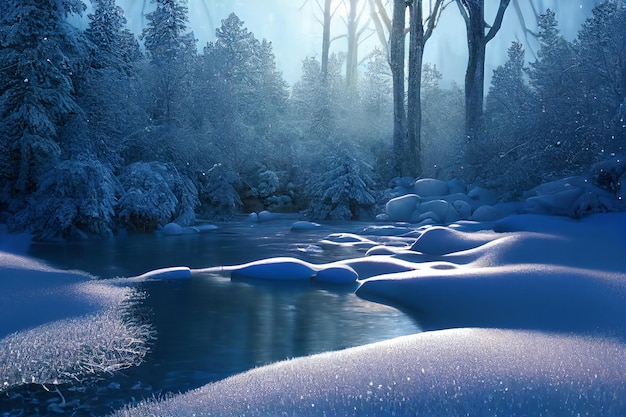An artistic photograph captures a serene winter solstice afternoon in the countryside, showcasing an enchanting winter wonderland. Snow blankets the entire landscape, forming thick, undisturbed layers on the ground, the tops of trees, and the branches, creating a pristine white carpet devoid of any footprints or markings. In the heart of the scene lies a small, free-moving pond or stream that appears to be almost frozen, with snow-covered rocks and gentle mounds of snow on its edges. Surrounding this water body are towering pine trees and older, leafless trees, cloaked heavily in snow, projecting a timeless, serene ambiance. A source of light, possibly the sun, casts a warm, golden glow from the background, illuminating the snow and creating a beautiful contrast against the slightly dull, wintry color scheme. This light, though warm, is insufficient to melt the snow, preserving the tranquil, unspoiled aura of the scene. The sky above is blue, enhancing the overall bright and tranquil atmosphere, while the landscape below remains a testament to the deep cold of the winter solstice.